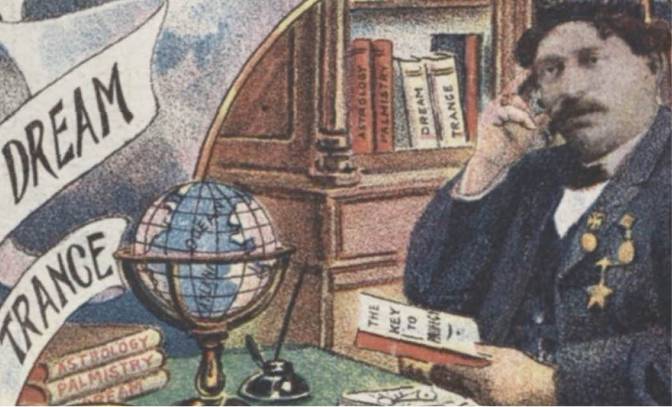This detailed image appears to be an old drawing of a Caucasian man seated at a desk, deeply in thought. The man has fairly pale skin, dark short hair, and a brown mustache. He is wearing a dark brown or black hat and an old-style suit adorned with three gold medals—two oval-shaped and one star-shaped—on the left breast. He holds a book in his left hand that reads "The Key To," with the last word remaining unclear. His right hand touches the side of his head, conveying a contemplative state. In front of him on the desk, there is a quill and inkwell, a globe, and three books titled "Astrology," "Palmistry," and "Dream." A wooden bookshelf in the background holds more books with the same titles. On the left side of the image, two banners in all capital letters read "DREAM" and "TRANCE," supplemented by the words "Astrobiology," "Palmistry," and "DREAM" again, emphasizing the themes of the illustration.